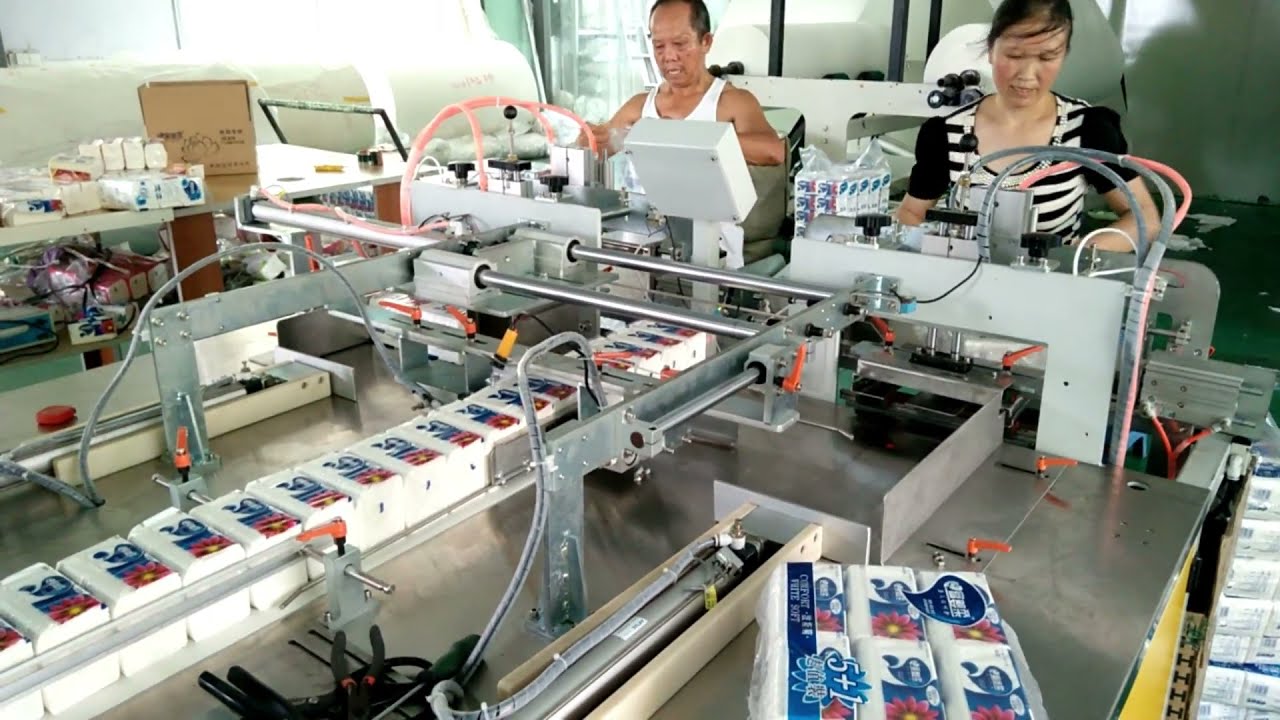This is a landscape-style color photograph taken inside a brightly lit factory specializing in the packaging of napkins or tissues. In the foreground, a sophisticated industrial packaging machine dominates the scene with its mélange of gray and stainless steel parts, adorned with buttons, tubing, and wiring. The machine features a white and silver console and a conveyor belt transporting neatly stacked packages of white napkins. To the right stands a woman with black hair, wearing a black-and-white striped blouse with black sleeves, intently focused on her work. To the left is a middle-aged, balding man with dark skin, donning a white tank top, equally absorbed in his task. Both workers are stationed at the machine which appears to require their dual operation. The setting includes a silver metal counter on the right, covered with additional packages and more on the floor around it. In the background, further tables support open packages and a brown box. The environment, marked by chrome table tops and sliding glass doors, is indicative of a bustling and organized packaging plant.